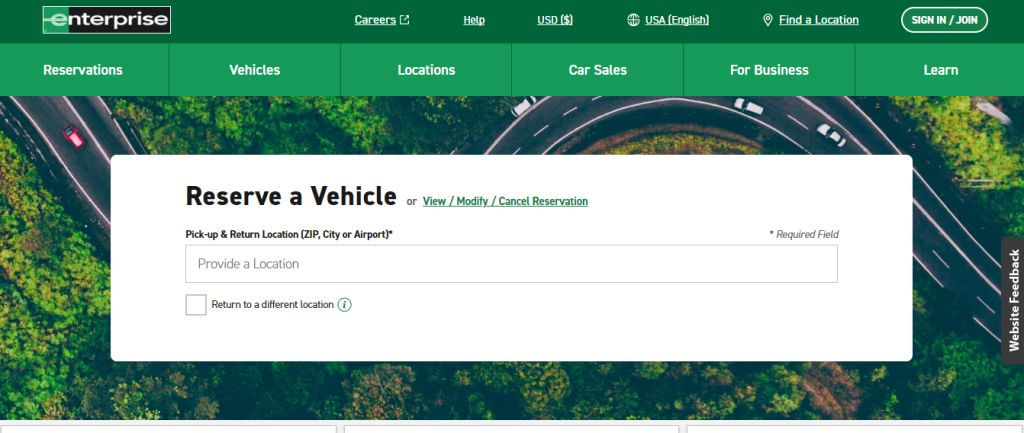This image showcases the Enterprise website's "Reserve Vehicle" page. The main window is dominated by a large, left-justified heading that reads "Reserve Vehicle." Adjacent to the right in smaller, green font are the options "View/Modify/Cancel Reservation."

Below this heading, the text prompts users to enter a "Pick-up and Return Location," with the instruction in parentheses indicating "zip, city, or airport" and a noticeable asterisk likely indicating required information. Beneath this prompt is a text input bar for users to enter their location details. Further down, there's a checkbox option labeled "Return to a different location," allowing users to specify a varied return point.

The background of the page features an image of a roadway filled with cars, subtly enhancing the theme of vehicular travel.